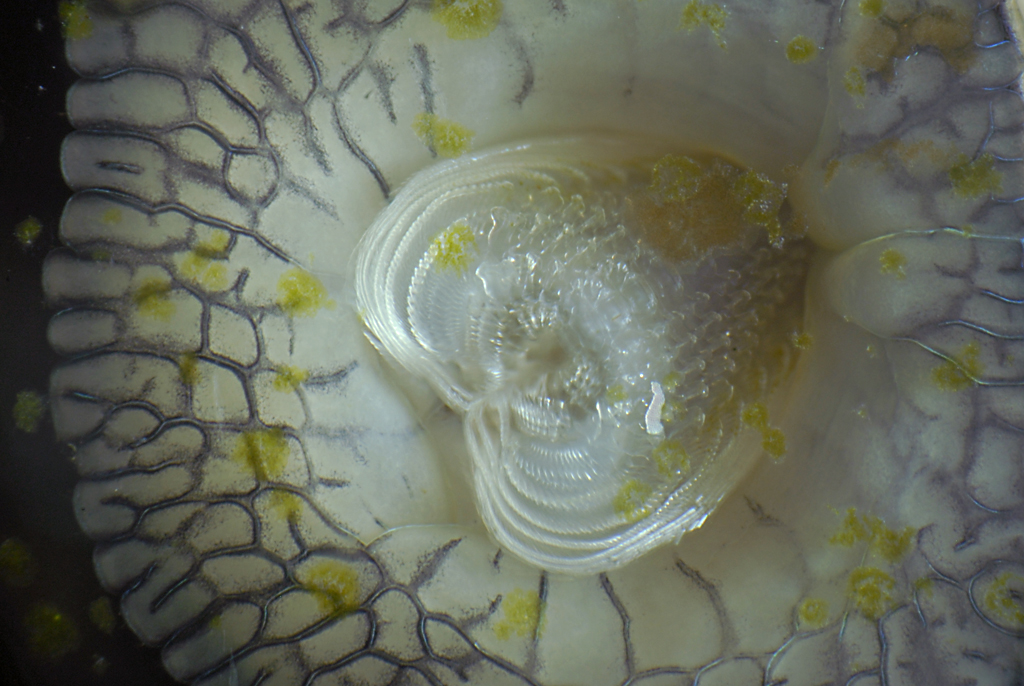The image depicts a highly detailed, potentially microscopic close-up of what could be a figurine or a biological structure such as the pistil of a flower. The central element is an upside-down, heart-shaped object with a mother-of-pearl sheen, featuring ripples and white dots. It is marked by an indention in the middle and is oriented to the right. Surrounding this heart-shaped structure is a bowl-like formation, primarily white, adorned with blue veins and interspersed with numerous yellow polka dots. The blue veins extend from the top to the bottom of the bowl and fan out in all directions. This intricate scene, with its vibrant color details and complex textures, evokes both an artistic and a naturalistic essence, making it appear like a harmonious blend of art and biology under close examination.